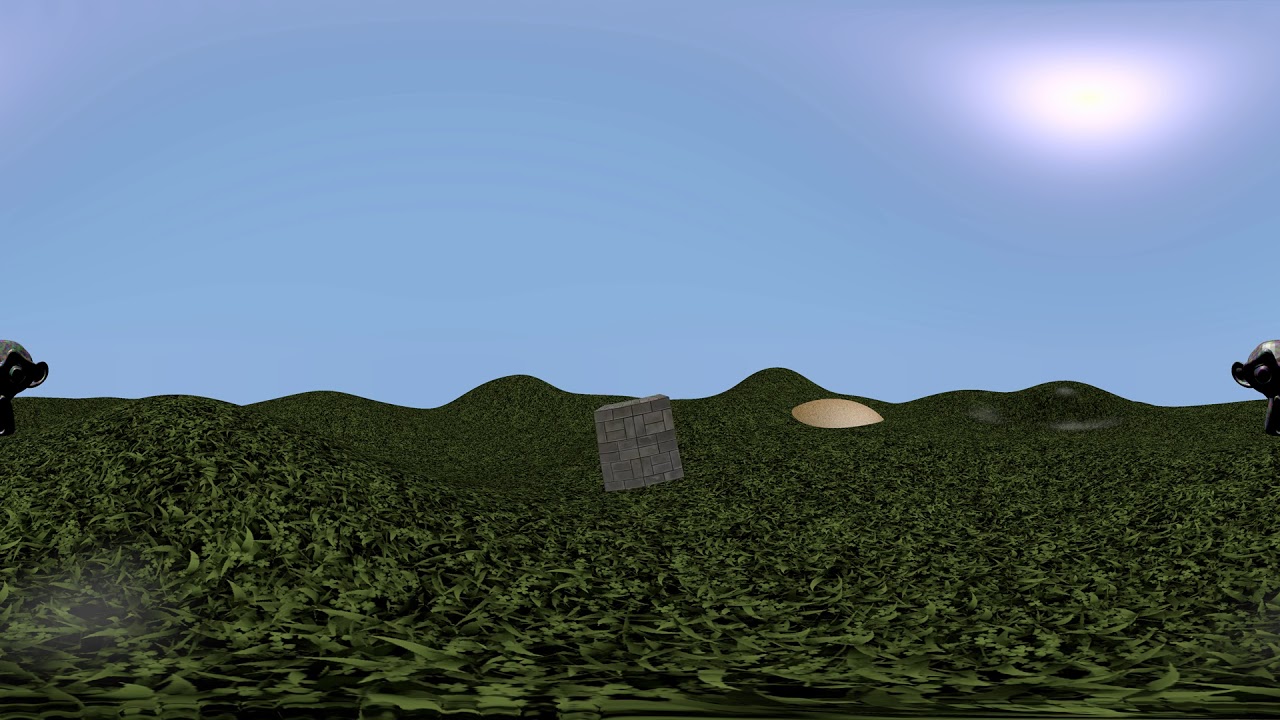The image portrays a CGI-rendered landscape with a grassy field in the foreground that resembles rolling hills drawn in dark green. In the center of the field, there is a slightly tilted gray cube composed of numerous smaller gray squares. Adjacent to it on the right side is a light yellow, bulbous dish-like object protruding from the ground. The background features a mostly light blue sky with the sun shining brightly in the top right corner. The sun is depicted with a white center and a pinkish periphery, emitting rays of white light. The scene includes additional elements: on the left and right edges, there are bulging forms that appear to be cartoon animal heads—one resembling a cow with a black nose, white face, and a white eye, and the other potentially a skunk. Toward the middle of the image, there are two large green mounds, between which the gray cube is situated, enhancing the surreal, virtual reality aesthetic of the picture.